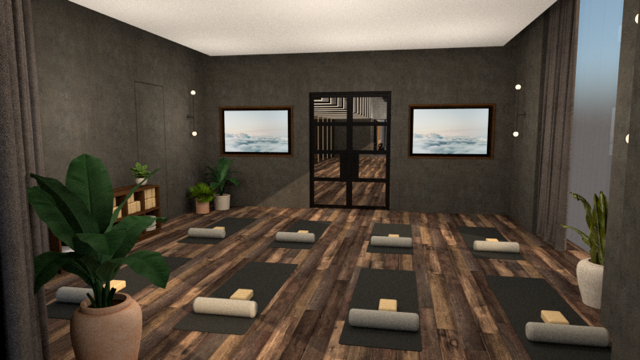This detailed digital rendering depicts the serene and minimalist interior of a yoga studio. The studio features rows of gray yoga mats, four per row, each equipped with a cylindrical bolster and a yellow block. The walls are painted a calming charcoal gray, contrasted by a pristine white ceiling and rustic wood plank flooring in varying shades of brown. Dark lighting enhances the tranquil ambiance.

On the walls, two TV monitors display relaxing images of clouds and the ocean, further promoting a soothing atmosphere. Circular lights are also installed on the walls, adding a soft illumination to the space. A large glass door with black borders is centrally located, reflecting parts of the room.

The studio is thoughtfully decorated with several potted plants, including one in a large white vase near a window with open curtains, allowing natural light to filter in. A wooden cabinet with some boxes on its shelves and an additional plant on top can also be seen. Above the cabinet, wall frames with paintings of the sky enclosed in brown frames add a touch of artistry to the environment. All these elements together create an inviting space designed for yoga, meditation, and other wellness activities.